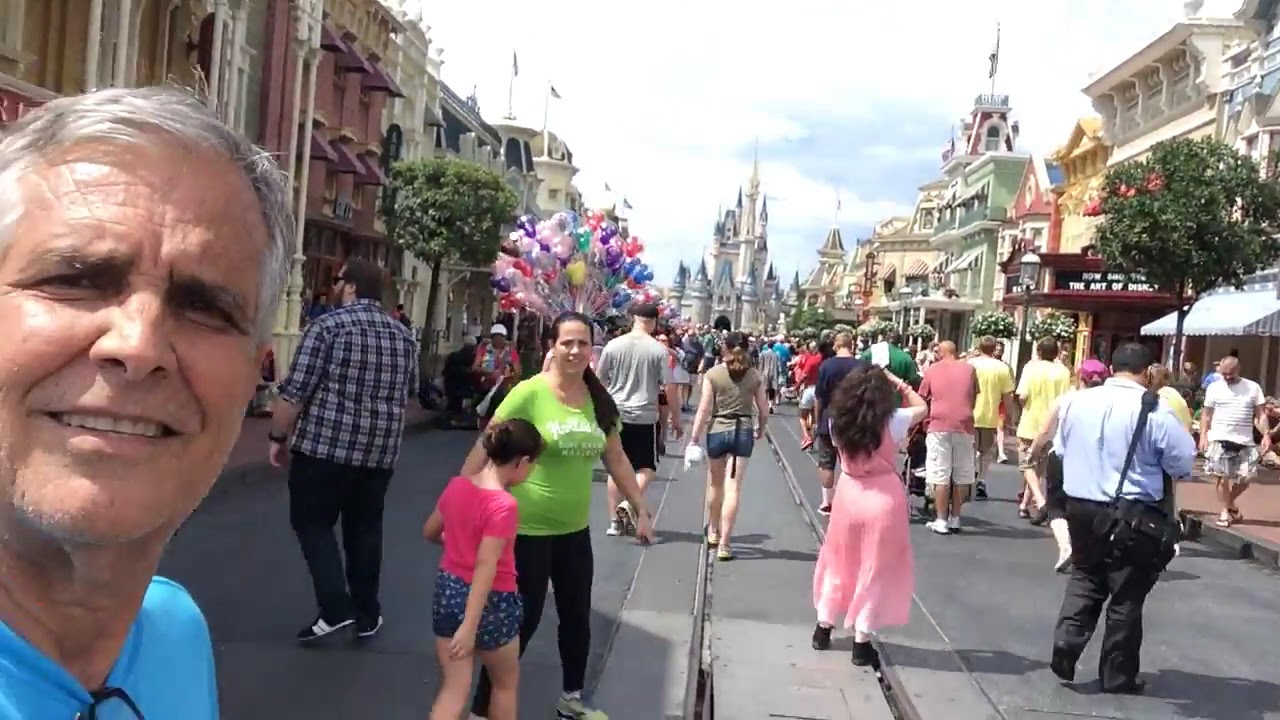The photo captures a bustling scene on Main Street at a Disney park, likely Disneyland or Disney World. At the street's horizon stands an iconic Disney castle under a bright blue sky scattered with white clouds. The street, lined with clusters of colorful buildings and verdant trees along the sidewalk, teems with around 30-40 people walking toward the castle. Trolley tracks run down the center of the street. 

Prominently, an older gentleman with short white hair and a light blue t-shirt stands on the left foreground, smiling and slightly squinting at the camera. Directly behind him, a woman in a green shirt is accompanied by a little girl wearing a pink shirt and blue shorts. To their left, a man in a plaid shirt and dark pants gazes at the surrounding attractions.

On the right-hand side, a lady in a pink jumpsuit and a man with gray pants and a white shirt walk among the crowd. Nearby, another man wearing a white t-shirt and shorts looks down as he walks. Scattered along both sides of the street, people sit at tables, and a large bouquet of balloons floats behind, adding to the vibrant atmosphere of the scene.